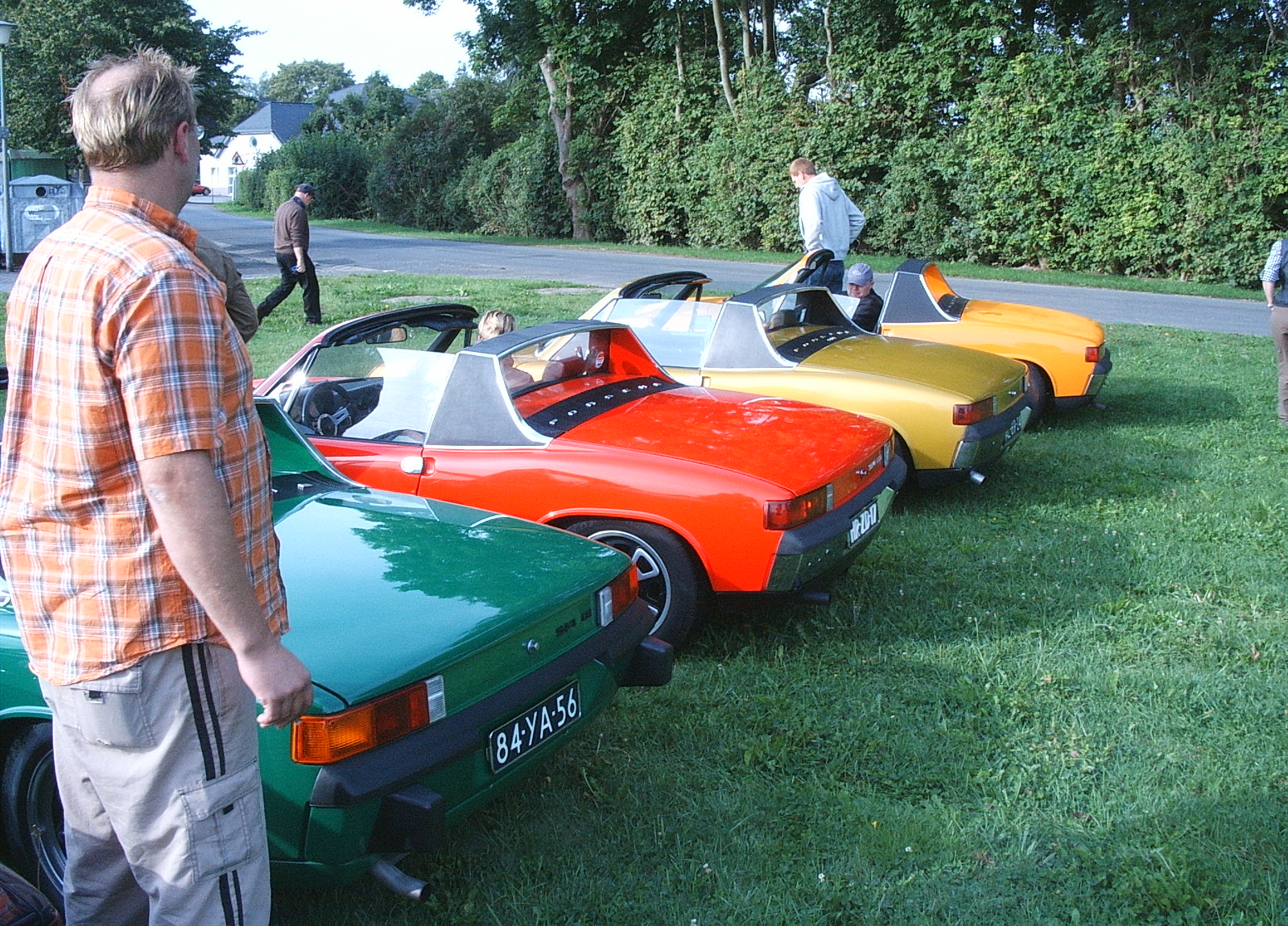The photograph depicts a sunny daytime scene with four small convertible sports cars arranged diagonally on a lush, grassy area filled with small white flowers. From left to right, the cars are dark green, dark orange, gold, and light orange. The back and side profiles of the cars are visible. 

Behind the grassy area lies a narrow, paved road lined with a dense row of trees. Closest to the viewer, a man wearing beige cargo pants, an orange and white plaid shirt, and glasses is standing beside the green car, partially obscuring its rear tire. The green car features a license plate reading "8 4 YA 5 6."

The dark orange car has a person seated in the passenger seat. In the light orange car, a man in a gray hoodie sits facing the camera. Another man, clad in gray pants and a gray hat, walks away from this car towards the road. Also visible is a person walking towards the road in front of the cars, contributing to this lively yet tranquil scene.